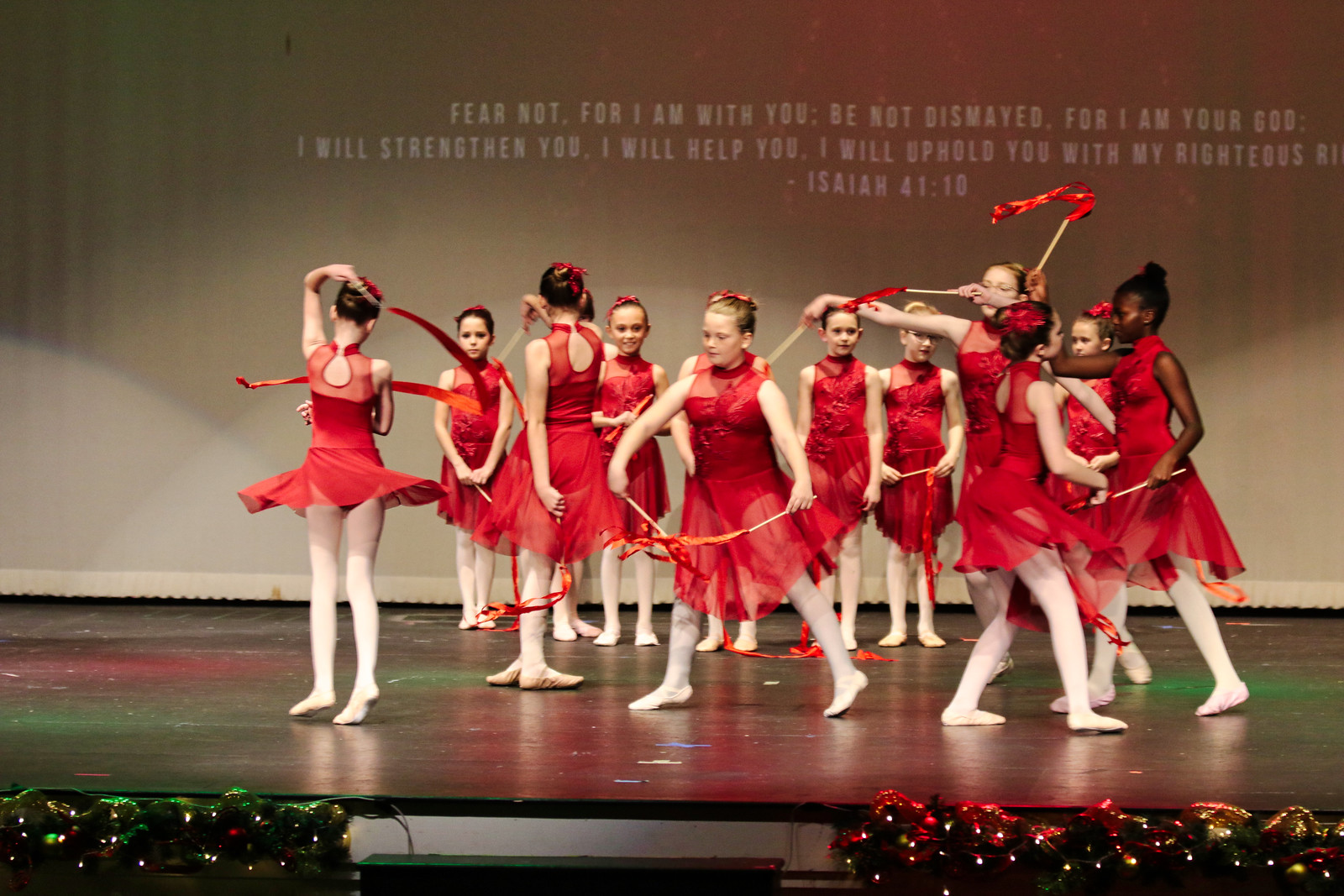The photograph captures a ballet recital featuring twelve 12 to 14-year-old girls performing on stage. All of the dancers are uniformly dressed in elegant red ballet outfits. These sleeveless dresses have a modest top and a tulle skirt that adds grace to their movements. Each dancer complements her attire with white leggings and tan ballet shoes, and their hair is meticulously pinned up into buns adorned with ribbons. Some of the girls are brandishing ribbon sticks of varying lengths and quantities—some wield one, while others hold two. The stage front is decorated with Christmas lights, adding a festive touch to the scene. Behind the dancers, a beige backdrop displays a projected biblical quote in white text: "Fear not, for I am with you. Be not dismayed, for I am your God. I will strengthen you. I will help you. I will uphold you with my righteous right," from Isaiah 41:10. The combination of the recital's visual appeal and the inspirational message suggests a celebration of Christian faith.